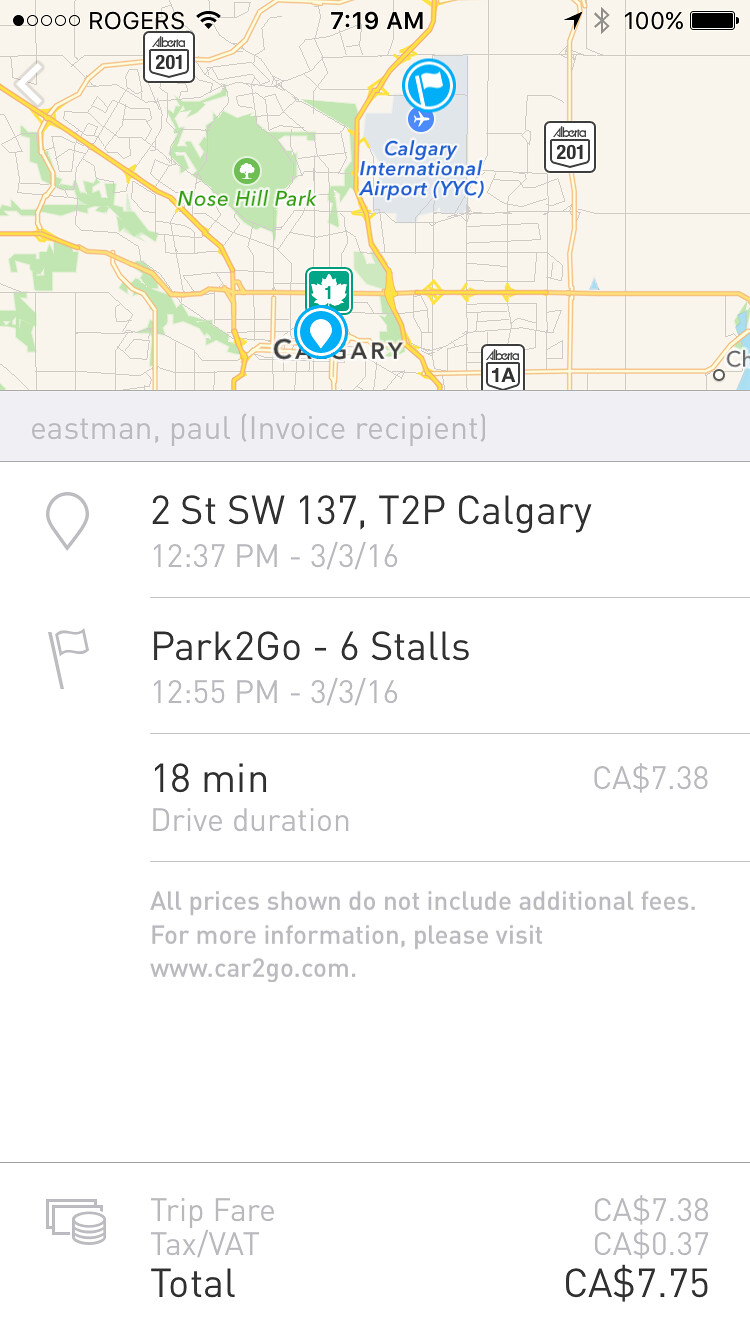This image appears to be a screenshot of an app on an iPhone showcasing a trip fare invoice and associated details. The top 25% of the screen displays a small map highlighting the Calgary International Airport in blue text with a little flag icon. Additionally, Nose Hill Park is labeled in green. At the top of the screen, the time is 7:19 AM and the battery is fully charged at 100%. The bottom 75% of the screen provides detailed trip information. The departure location is 2 Street Southwest 137, T2P, Calgary, and the final destination is Park To Go with 6 stalls. The trip lasted 18 minutes and is listed to cost CA $7.38, with an additional tax/VAT of CA $0.37, bringing the total to CA $7.75. It's noted that all prices shown do not include additional fees, and more information can be found at www.cartogo.com. The invoice recipient is Eastman Paul. The dates and times further illustrate the timeline of the trip, with specific mentions of activities at 12:37 PM and 12:55 PM on March 3, 2016.